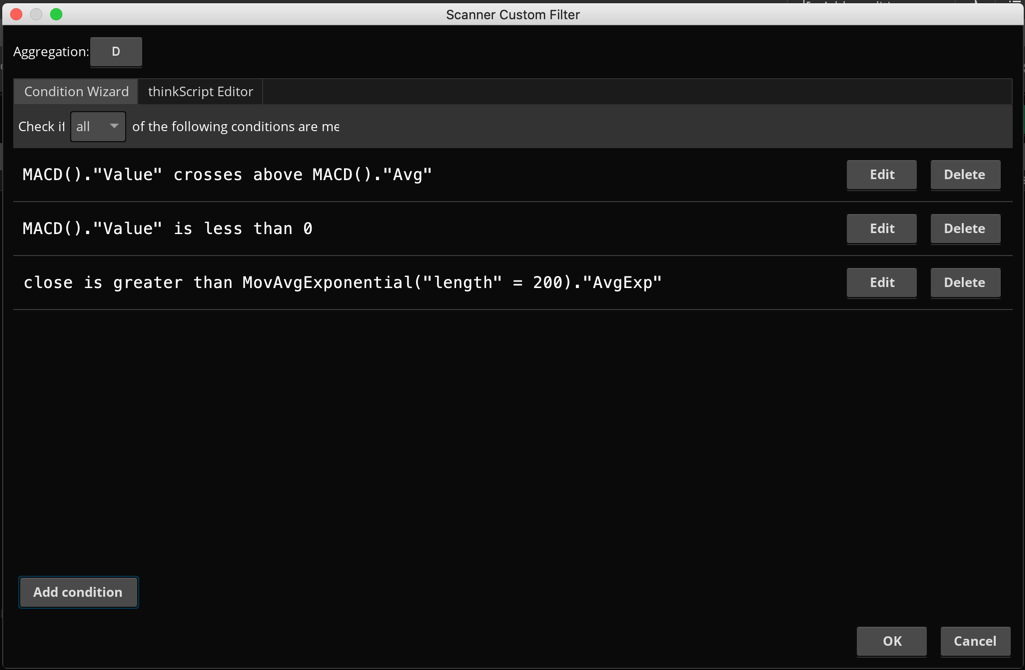The image displays an interface header prominently featuring the title "Scanner Custom Filter" in black, centered against a light gray background. On the top-left corner is a filled red dot, with a gray dot in the middle, and a green dot on the far right.

Below the header, the interface consists of a window with a black background. In the upper left of this window, the label "Aggregation:" appears in white. Adjacent to this is a medium gray rectangle with the letter "D" in white text at its center. Further to the right, a lighter gray rectangular icon displays the text "Condition Wizard" in white.

Continuing to the right, the interface transitions into a darker gray background. The text "thinkScript Editor" is displayed here in white, with a capital 'S' in "thinkScript". Directly beneath this section, a quasi-3D header area is visible with the label "Check it" in white on the left. A dropdown menu, featuring a light gray background and white text, indicates the option "All." Another phrase in white text reads "of the following conditions are ME," which is partially cut off.

The interface reverts to a black background, displaying a complex formula in white font: "MACD (.) 'value' crosses above 'MACD (.) 'AVG'." To the right of this, two medium gray rectangular buttons are visible, labeled "Edit" and "Delete" in white text respectively.

At the interface's bottom left, a medium gray rectangular button labeled "Add Condition" in bold white text stands out. The bottom right corner houses two smaller gray rectangular icons, one saying "OK" on the left and the other "Cancel" on the right, both in white writing.